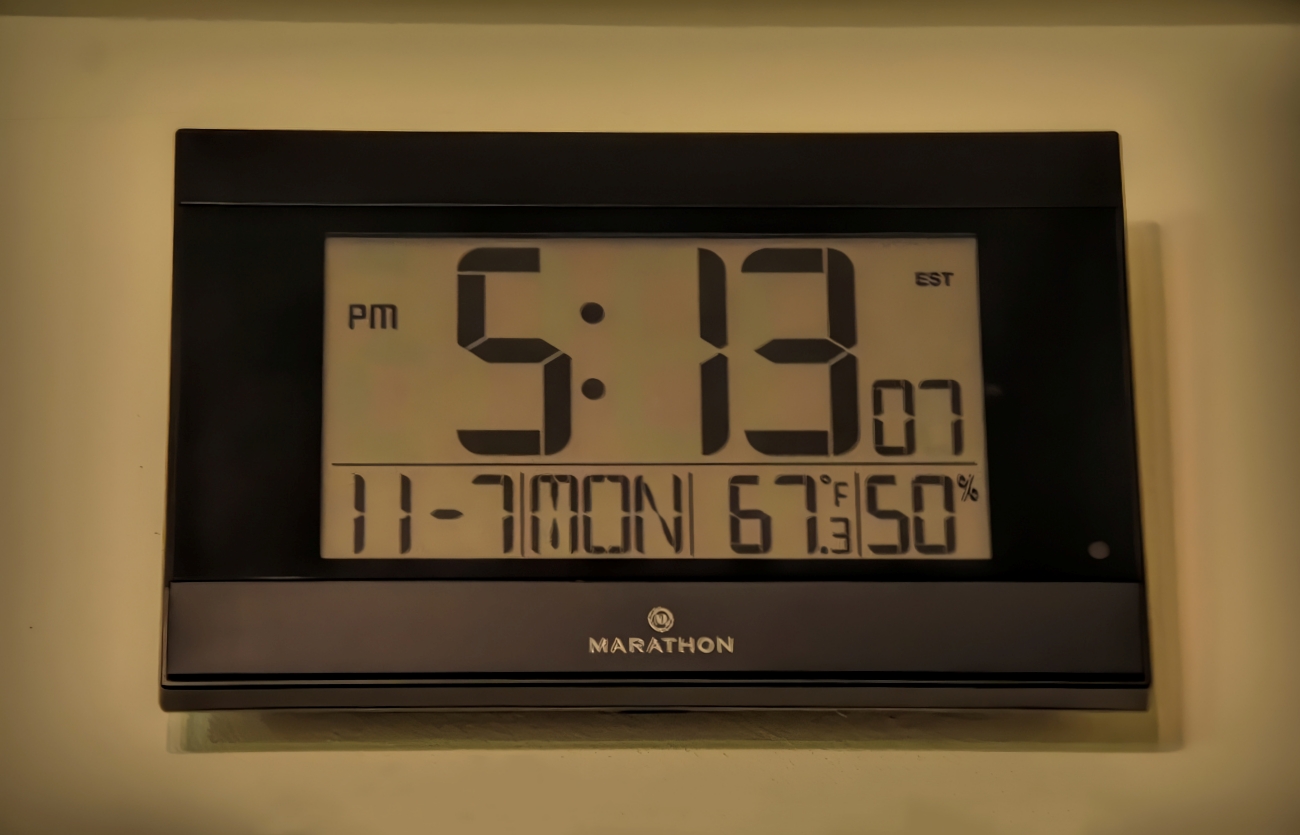The image depicts a digital clock displaying the time as 5:13:07 PM, signified by the 'PM' indication and 'ESP' notation for Eastern Standard Time on the right side of the clock face. The clock features a clear background and black digits, encased in a black plastic frame. Below the main time display, a secondary row provides additional information: the date as November 7th (11.7), the day as Monday, the temperature as 67.3 degrees Fahrenheit, and the humidity level at 50%. At the very bottom of the clock, the text reads "Marathon," suggesting the clock's brand. The clock appears to be lying on its back on a slightly yellow surface, implying it is not mounted on a wall. The lighting suggests that the room is illuminated by ambient evening light, hinting that the clock face might light up at night.